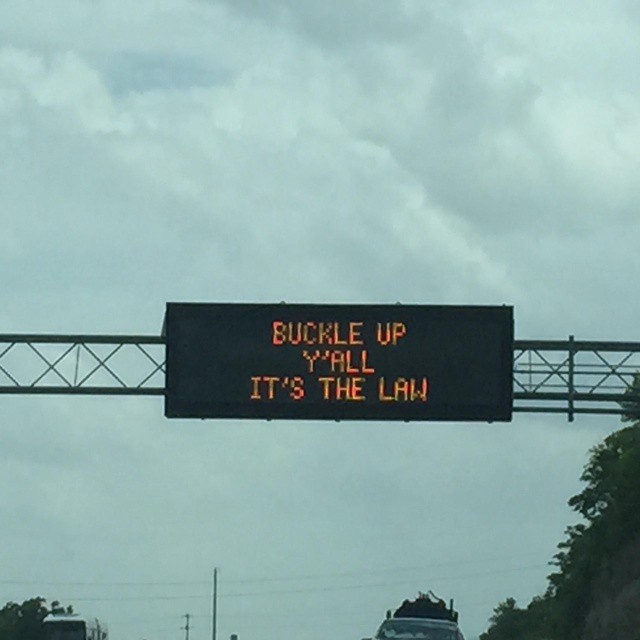The image captures a large roadside sign suspended over a highway, likely in Texas, based on the colloquial language used. The sign, displayed in orange text on a black background, reads, "Buckle up, y'all, it's the law," and serves as a public service announcement emphasizing the importance of wearing seatbelts while driving. The sign is mounted on a metal grating that spans the width of the highway, and below it, faint traces of a car are visible. The background features a cloudy, gray sky with power lines and a hint of trees to the right, further highlighting the sign as the focal point of the image. The message is particularly apt given the context of being on a highway, reinforcing the necessity of seatbelt safety.